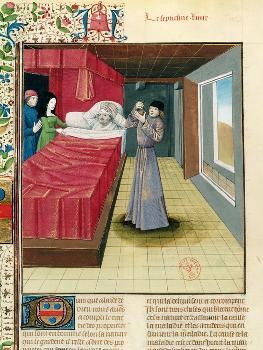This small, intricate photograph, seemingly taken from a book or magazine, features a detailed and vibrant artwork of four individuals in a room. The page is light brown with elaborate floral and decorative decals running along the left side and partially across the top. Despite the text above and below the image being illegible, the main focus is a scene centered on a sickly man lying in a bed adorned with a red cover. Standing beside him are two women; one with dark hair in a green dress, facing the camera with her hands on her head, and another man in a blue shirt behind her. The room itself has a blue wall with a prominently seen red accent on the left and a yellow floor. On the right side of the bed, there is an individual in a long blue dress, wearing a black hat, standing beside an open window. This person appears to be a doctor, holding and examining a bottle or potion, looking intently at the contents. The overall scene conveys a moment of care and concern within a visually rich and detailed setting.